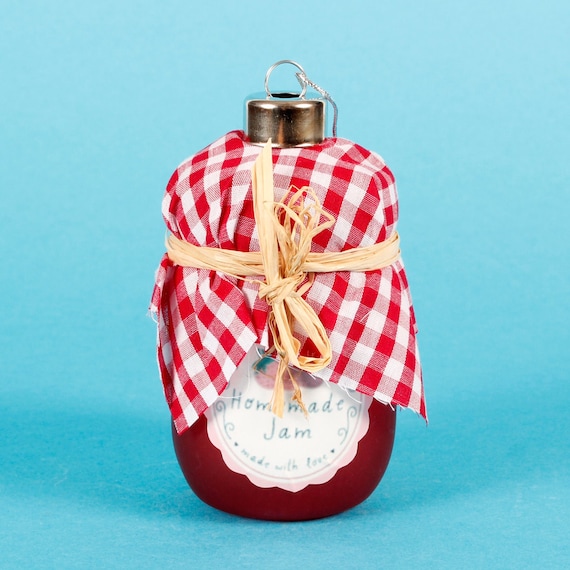This image presents a tall, rectangular photo with a baby blue background and prominently features a jar of homemade jam. The jar is adorned with a red and white checkered gingham cloth atop, fastened loosely with a straw-like raffia ribbon tied in a vertical bow. The jar itself is capped with a unique metal lid equipped with a circular stopper, possibly for added freshness. Below the decorative cloth, the jar flaunts a white label reading "Homemade Jam – Made with Love," complemented by an image of a strawberry. The jam inside is a rich, dark red, suggesting a luscious, berry-filled preserve.